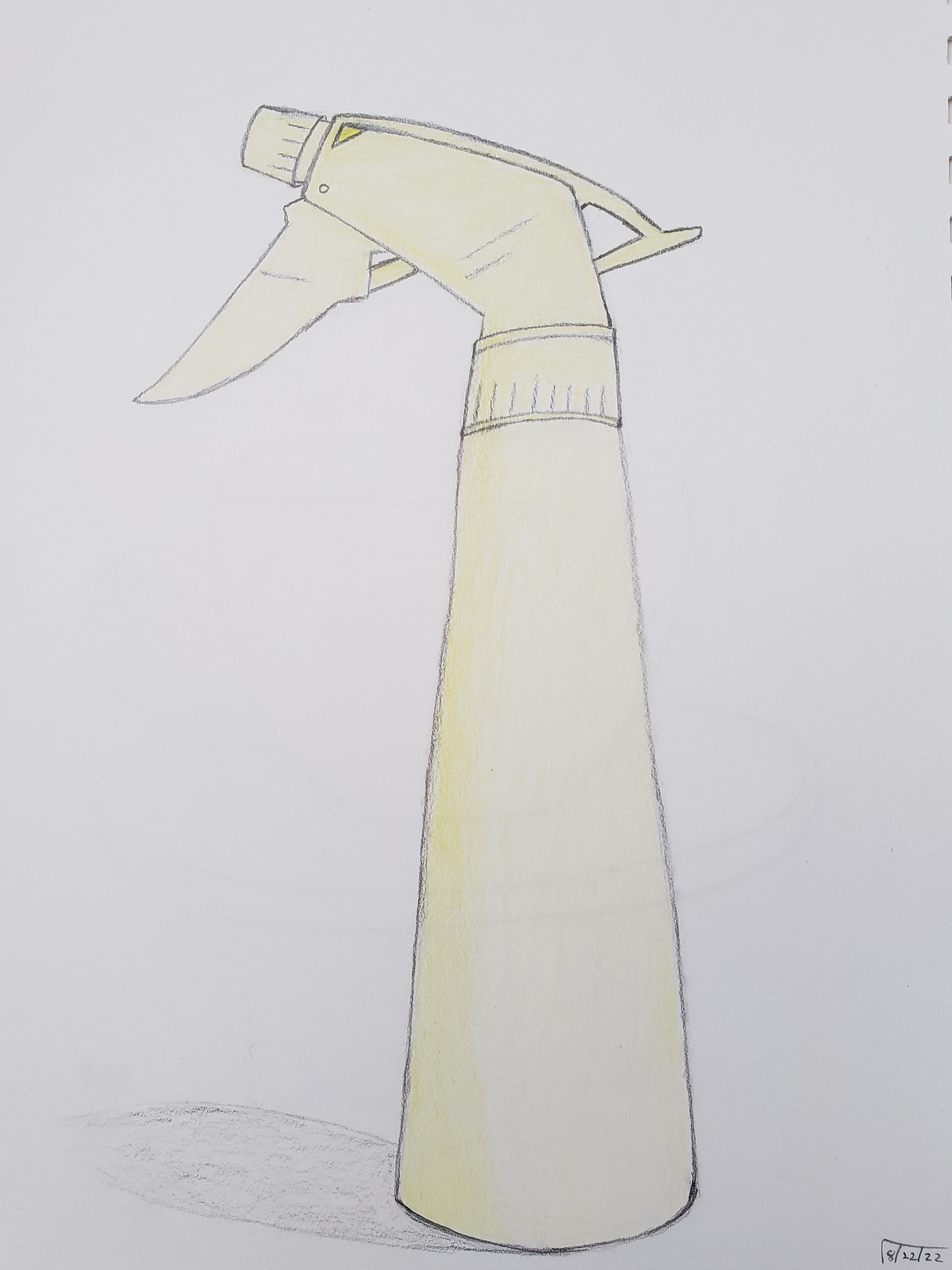This image is a detailed hand-drawn illustration of a spray bottle, rendered on what appears to be grayish paper using colored pencils or crayons. The spray bottle is primarily white with a slight yellowish tinge and does not seem transparent. It has a somewhat tall, cylindrical shape, reminiscent of a paper towel roll or a thin beer bottle. The bottle narrows as it ascends, similar to the end of a baseball bat, leading up to a spray handle at the top, which is also white with notched detailing. The handle features a prominent button designed to be pressed to activate the spraying mechanism. A notable detail in this drawing is a timestamp located in the bottom right corner, reading either "9-12-22" or "82222," potentially indicating the date the illustration was created. A subtle black shadow beneath the bottle adds depth to the image, enhancing its realistic appearance.